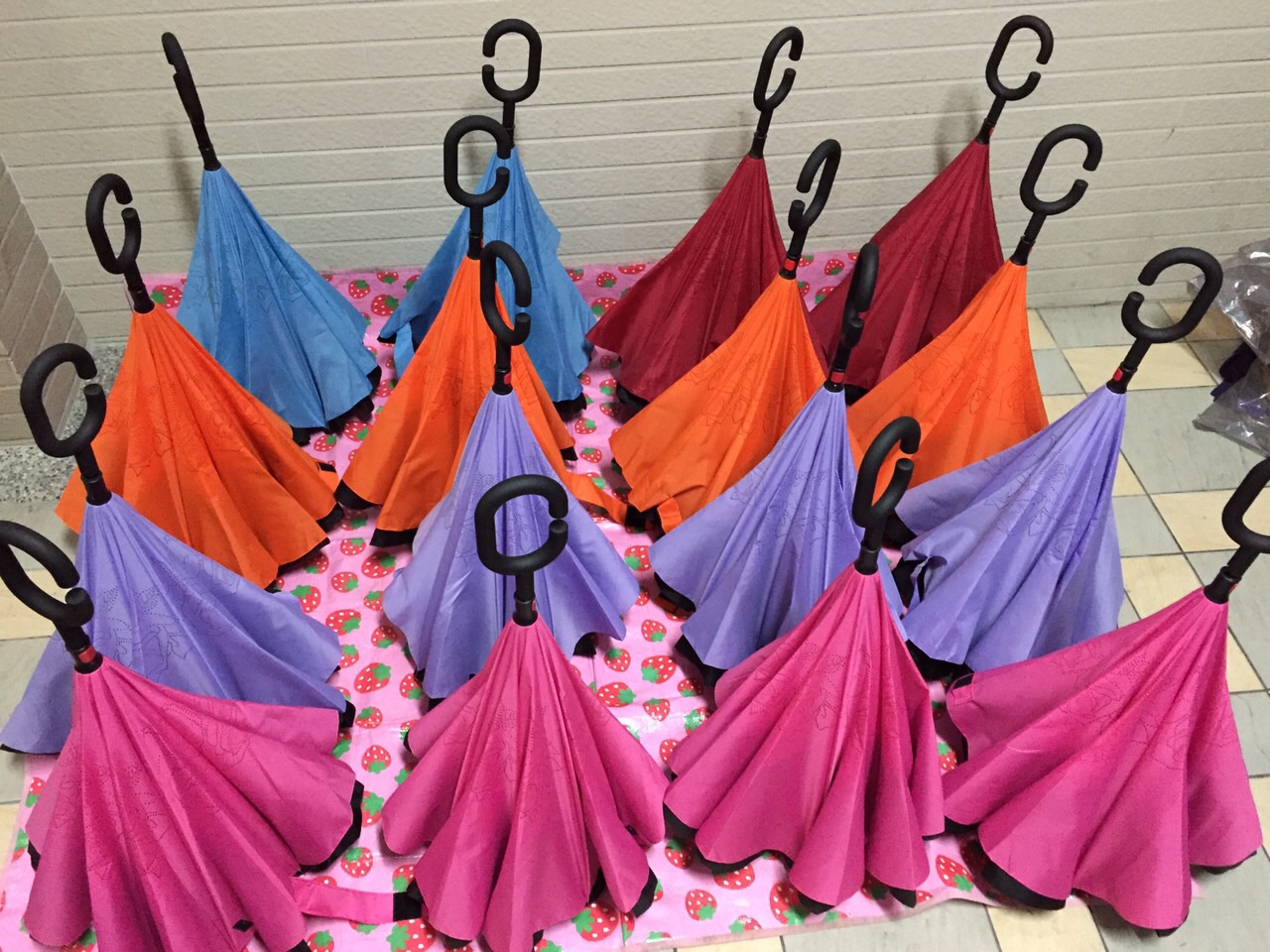The image depicts a room with white brick walls and a light blue and white checkered floor, featuring an arrangement of 16 identical objects on a pink tablecloth patterned with cartoon-like strawberries. The objects resemble mini tents or upside-down umbrellas, each with a black plastic C-shaped handle protruding from the top. These items are organized in a grid of four rows and four columns. The first row at the front consists of pink objects. The second row features lavender or blue objects. The third row consists of orange objects, and the final row has two turquoise objects on the left and two crimson objects on the right. The pink strawberry tablecloth is spread out on the floor against a white painted wall with visible lines.